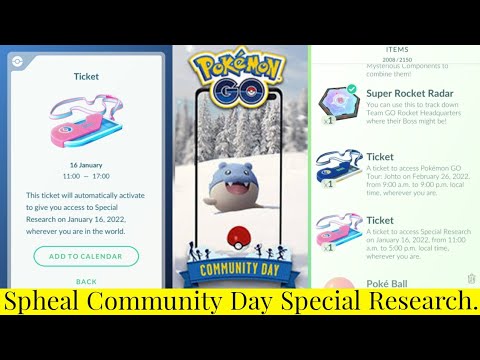This image is a promotional screenshot for a Pokémon GO event, specifically a Community Day focused on the Pokémon Spheal. Prominently featured is the iconic Pokémon logo with its signature yellow font outlined in blue, followed by the word "GO", which includes a Pokéball in the middle of the "O". The background depicts a snowy landscape with snow-covered trees, fitting for the Pokémon Spheal, which is pictured sitting on the snow.

The image highlights information about a Community Day event scheduled for January 16th, 2022, from 11:00 to 17:00. It mentions a ticket that automatically activates to grant access to special research on that date, available globally. "Add to Calendar" is emphasized in a green oval, encouraging players to mark their calendars. The text also notes items and bonuses available from 2008-2150, including a Super Rocket Radar which can be used to find the Team GO Rocket Headquarters and its boss.

The overall design of the image suggests it is a brochure, divided into three columns with small font text explaining event details, activities, and special items associated with the Spheal Community Day.